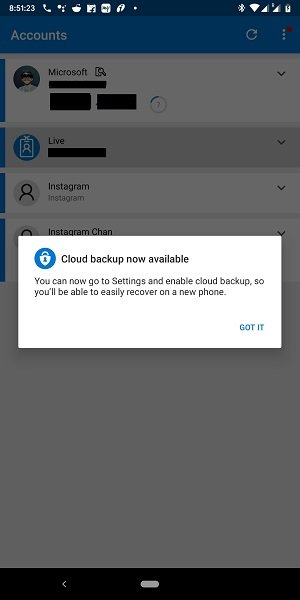The screenshot features a smartphone interface, capturing the top status bar and part of a settings menu. At the top, the navy blue status bar displays the time, "8:51," alongside several white icons: a phone, various circles, a small robot head (potentially Android's mascot), two overlapping squares, the Facebook icon, a dot, the Bluetooth symbol, the Wi-Fi signal, two signal strength indicators, and a battery icon.

Below this, the interface transitions into a grayed-out background, possibly indicating a settings menu. The top section showcases a tab highlighted in white and blue with the word "Accounts" in white font, accompanied by a refresh icon and three white dots with a red notification dot.

Further down, a white box presents a header with a man's photo labeled "Microsoft" in black text, accompanied by an icon symbolizing a document with a magnifying glass. Below this header, there are three areas obscured in black, presumably censoring sensitive privacy information. A blue and white circular icon and a pull-down tab follow.

The next section highlights another blue and white circular icon labeled "Live," with an adjacent black privacy bar, followed by another pull-down tab.

Continuing, there is another white box. This segment features a gray circle with an abstract cartoon figure, labeled "Instagram." It includes a down arrow and repeats the word "Instagram" next to "Sean," with another cartoon icon and a pull-down arrow.

In the middle of this interface, a pop-up notification with a blue and white padlock icon announces, "Cloud backup now available" in black text. It advises enabling cloud backup in settings to facilitate easier recovery on a new phone. The notification concludes with a blue "Got it" button.

At the bottom of the screenshot, there's a black tab with a white back arrow and a gray line.